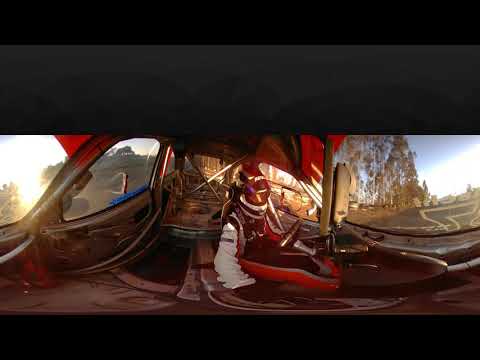The image captures the interior of a race car, showcasing a driver who is actively engaged in steering the vehicle. The driver, positioned in the stripped-down cockpit, is garbed in a distinctive racing suit that features red stripes along the sides, black around the midsection, and white sleeves, complemented by matching gloves. The helmet, a sleek black and white with a visor covering the face, further indicates the high-speed nature of the activity. The vehicle is designed for performance, evident from the minimalist interior and visible roll cages behind the driver. The surrounding scenery, visible through the car’s windows, includes a tree-lined street under a bright blue sky with scattered clouds. The sun shines intensely from the left, highlighting the dynamic environment. An orange roof canopy adds a splash of vibrancy to the scene, while outside, the pavement, possibly marked with the number 7, stretches out with hints of distant buildings and grassy patches.